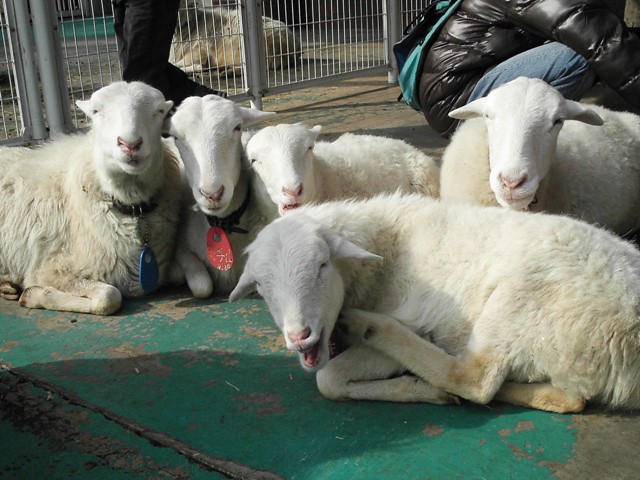This detailed photograph captures five freshly sheared white sheep laying on a worn, teal-painted concrete floor in an enclosure that resembles an animal petting zoo. The sheep, appearing to smile, are positioned with one in the foreground on the right, possibly itching its head with its back foot. It faces the camera directly, while the other four are lined up behind it, also facing the camera. Distinguishing features include two sheep on the far left wearing brown collars; one with a blue tag, the other with a red oval tag. The background reveals a gray metal gate, beyond which another sheep is lying down. To the right, a woman in a black puffy jacket and blue jeans is crouched down, seemingly attending to something on the ground, and further left, a pair of black-clad legs can be seen walking past the gate. The scene is a blend of animal interaction and human presence, creating a calm yet animated atmosphere.